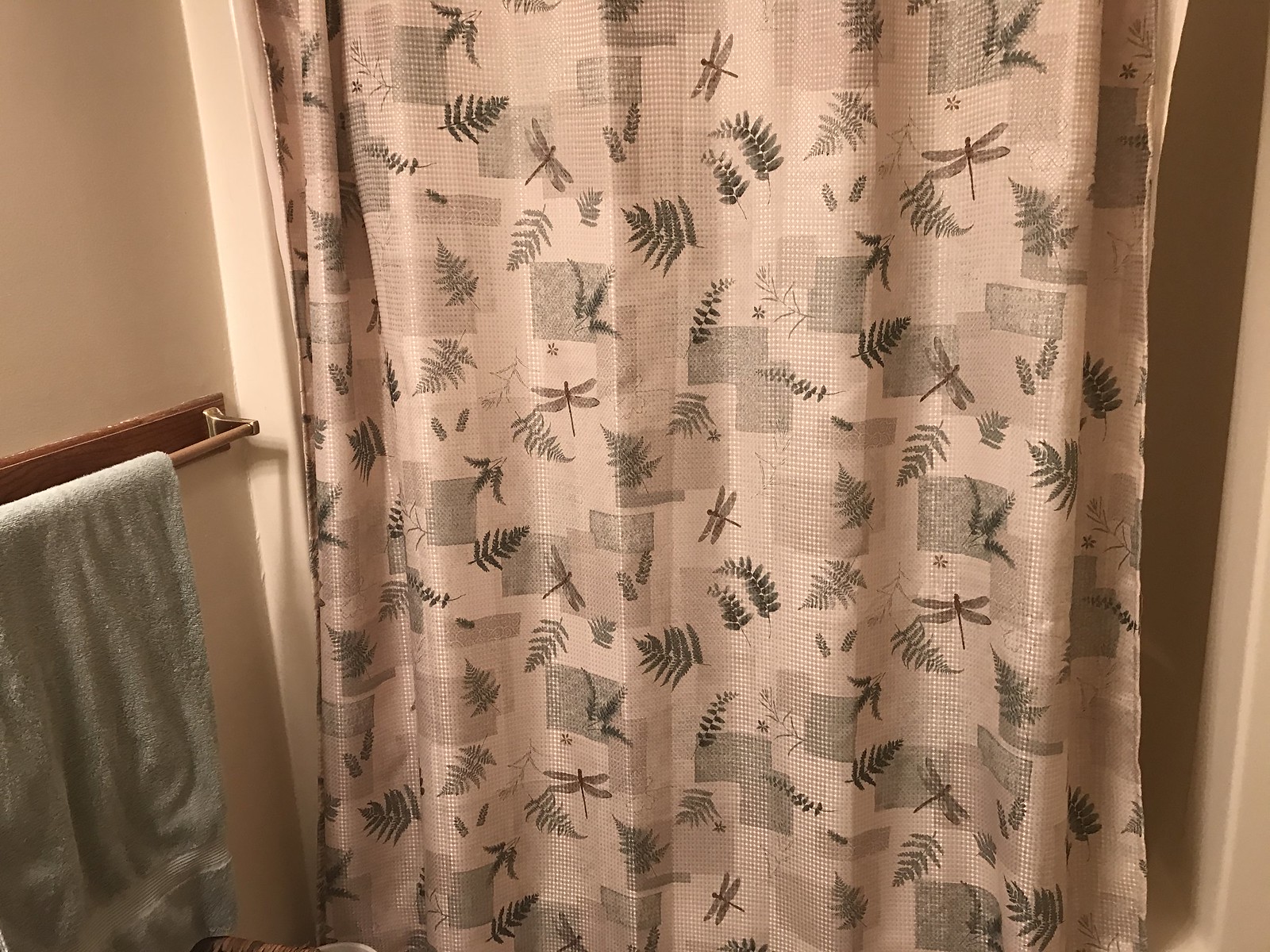This photo captures a detailed scene in a bathroom. Dominating the frame is a white shower curtain adorned with an array of designs. The curtain features a random pattern of dark and light gray squares interspersed with sketches of various leaves, including fern and maple leaves, as well as dragonflies. On the left side of the image, a brown, slender towel holder is visible, holding a blue towel against a wooden platform. The shower area itself has a porcelain edge that protrudes outward, and the interior of the shower is relatively dark, obscured by the curtain. A subtle shadow of the shower curtain is seen on the right side, hinting at the light conditions within the room.